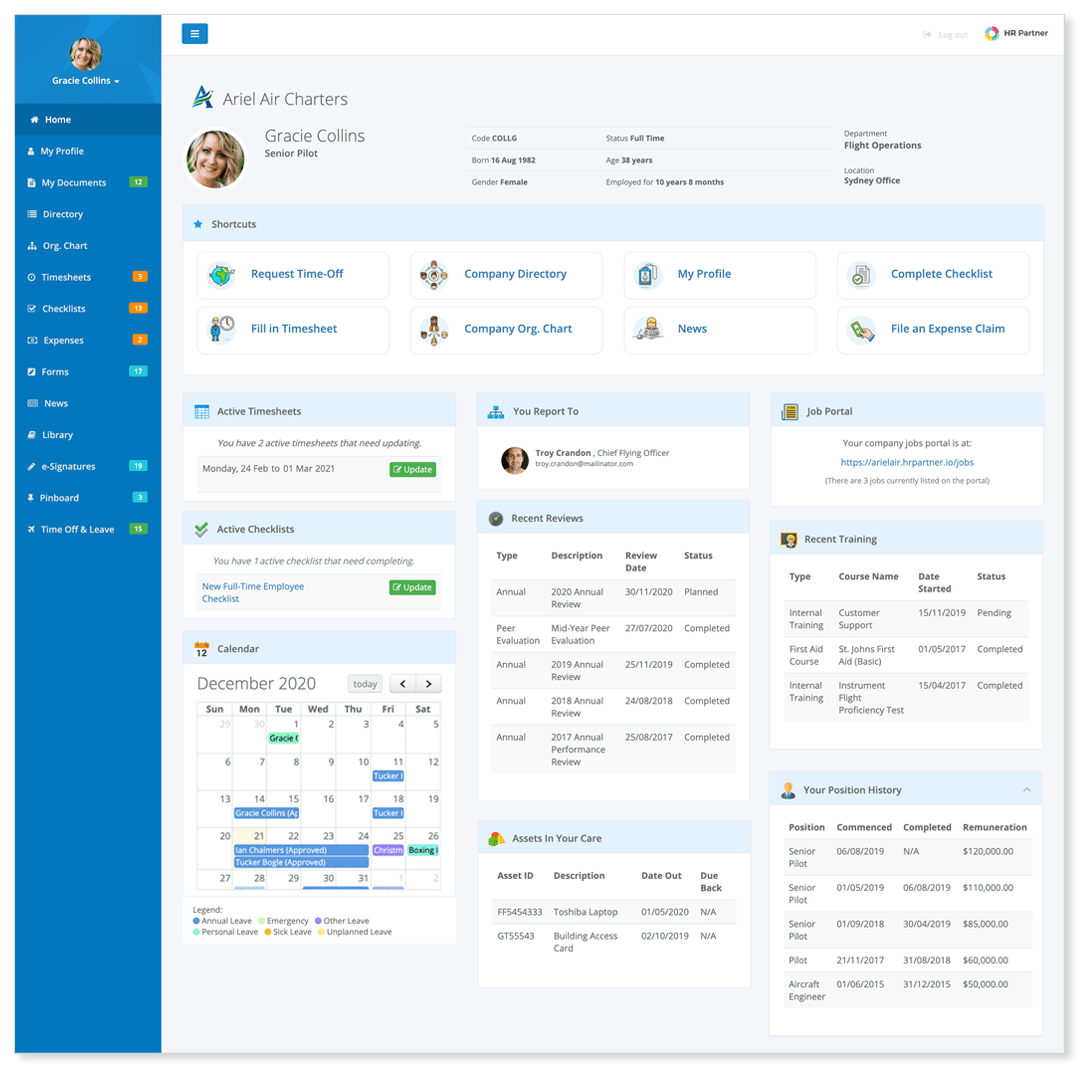The image is a detailed screenshot of a dashboard for "Aerial Air Charters." At the top, it displays the title "Gracie Collins, Senior Pilot." Below this header, various demographic fields are outlined. They include:

- Birth date: August 16th, year not fully visible (appears to be 19--).
- Gender: Female.
- Age: Possibly 58 or 38 years.
- Employment status: Full-time.
- Duration of employment: 10 years and 8 months.

The dashboard also features shortcuts for various functions, such as:

- Request Time Off
- Company Directory
- My Profile
- Complete Checklist
- Fill-in Timesheet
- Company Org Chart
- News
- File an Expense Claim.

In the middle section of the dashboard, it indicates that Gracie Collins reports to Troy Crandon.